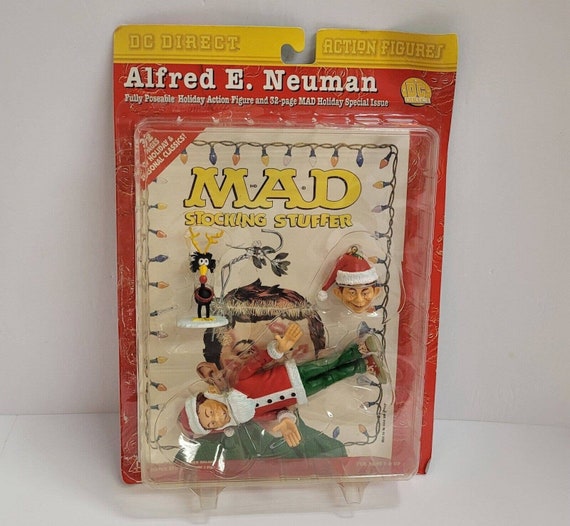The image depicts a display case on a white table with a white background. At the top of the clear plastic packaging is a yellow banner that reads "DC Direct Action Figures." Below this banner, the package is predominantly red and includes the white text "Alfred E. Newman," "Fully Posable Holiday Action Figure," and "32-page MAD Holiday Special Issue." Inside, you can see a MAD magazine labeled "MAD Stocking Stuffer" in yellow with decorative lights around it. The action figure of Alfred E. Newman, dressed as an elf with a Santa hat, red Santa top, and green leggings, is lying diagonally in the package. Additional items include a separate head of Alfred E. Newman wearing a Santa hat and what appears to be a black bird. The overall package shows some wear, appearing slightly bent. This collectible item evokes a sense of nostalgia, reminiscent of holiday stocking stuffers from the past.